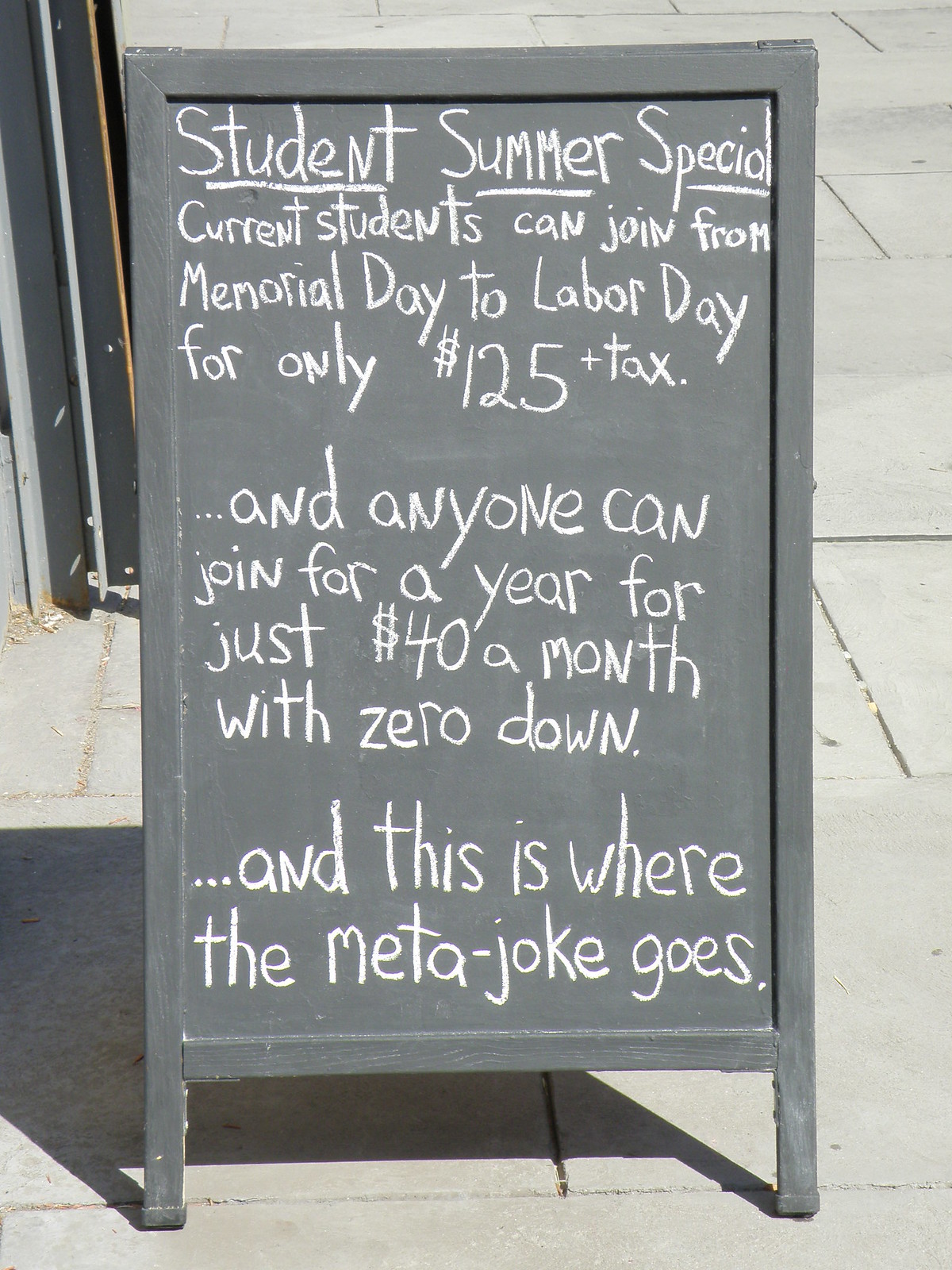This image depicts a gray wooden A-frame chalkboard sign positioned on a concrete sidewalk under bright sunlight, evidenced by the strong shadow cast on the street behind it. In white chalk, the sign prominently features an underlined header that reads, "Student Summer Special." Below this, it details two promotional offers: current students can participate from Memorial Day to Labor Day for $125 plus tax, and anyone can join for a year at a rate of $40 per month with zero down. The text concludes with, "And this is where the meta-joke goes." The background includes a doorway, but the focus remains solely on the sign and its vivid chalk-written message.